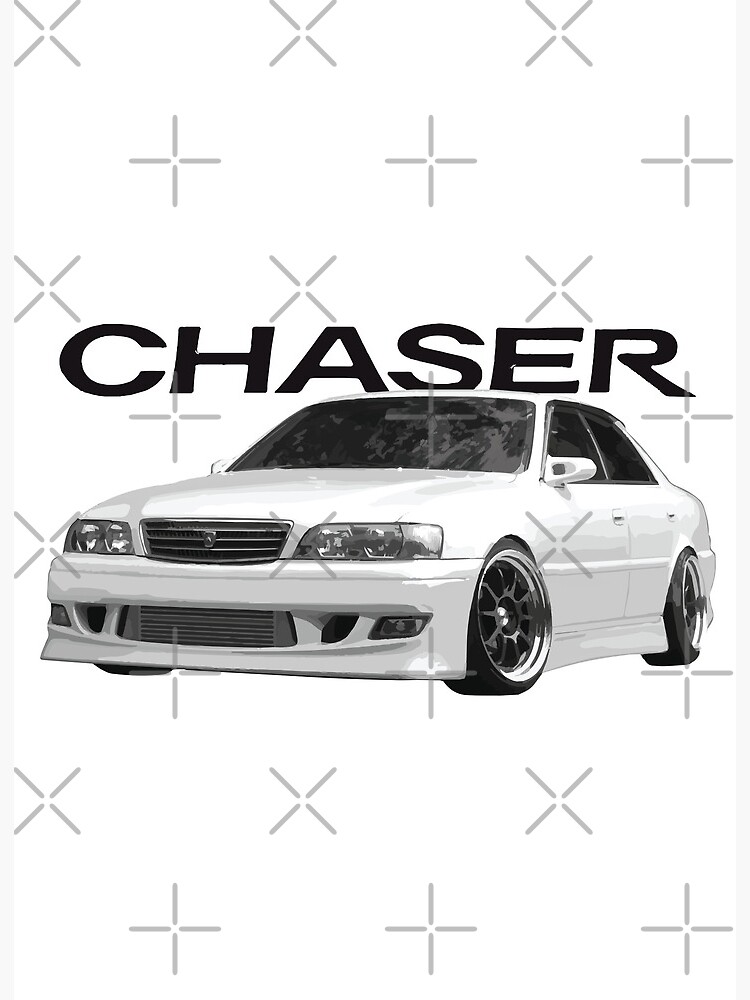This image appears to be a detailed graphic illustration of a white sedan, branded as "Chaser" in prominent black text across the top. The car, which resembles a luxury model possibly akin to a BMW, features sleek low-profile tires, shiny rims, and darkened windows. Additional sporty elements include a small front spoiler and a potential sunroof. The car's design is accented by black windshields and side mirrors, along with visible door handles indicating it is a four-door model. The entire artwork is overlaid with a pattern of silhouetted gray Xs and plus signs, adding a complex watermark effect that covers the background and stretches across the entire image.